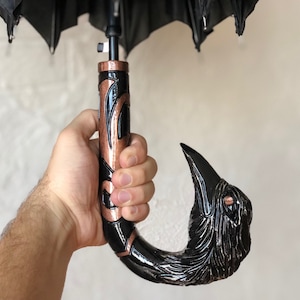In this image, a man holds an ornate umbrella against a cream-colored background. The black canopy of the umbrella is only partially visible at the top of the picture, revealing just the ends of the steel rods. The focus, however, is on the elaborate handle of the umbrella held in the man's left hand, positioned towards the bottom left of the image. The handle forms a large J shape, beginning as a blackened bronze or wood which features intricate gold or bronze design patterns. It transitions into a bird's head, complete with detailed engravings resembling feathers, and highlights of white and bronze or gold accents. The bird's head, primarily black, has a prominent eye that appears to be made of gold or bronze, adding to the umbrella's luxurious and intricate design.